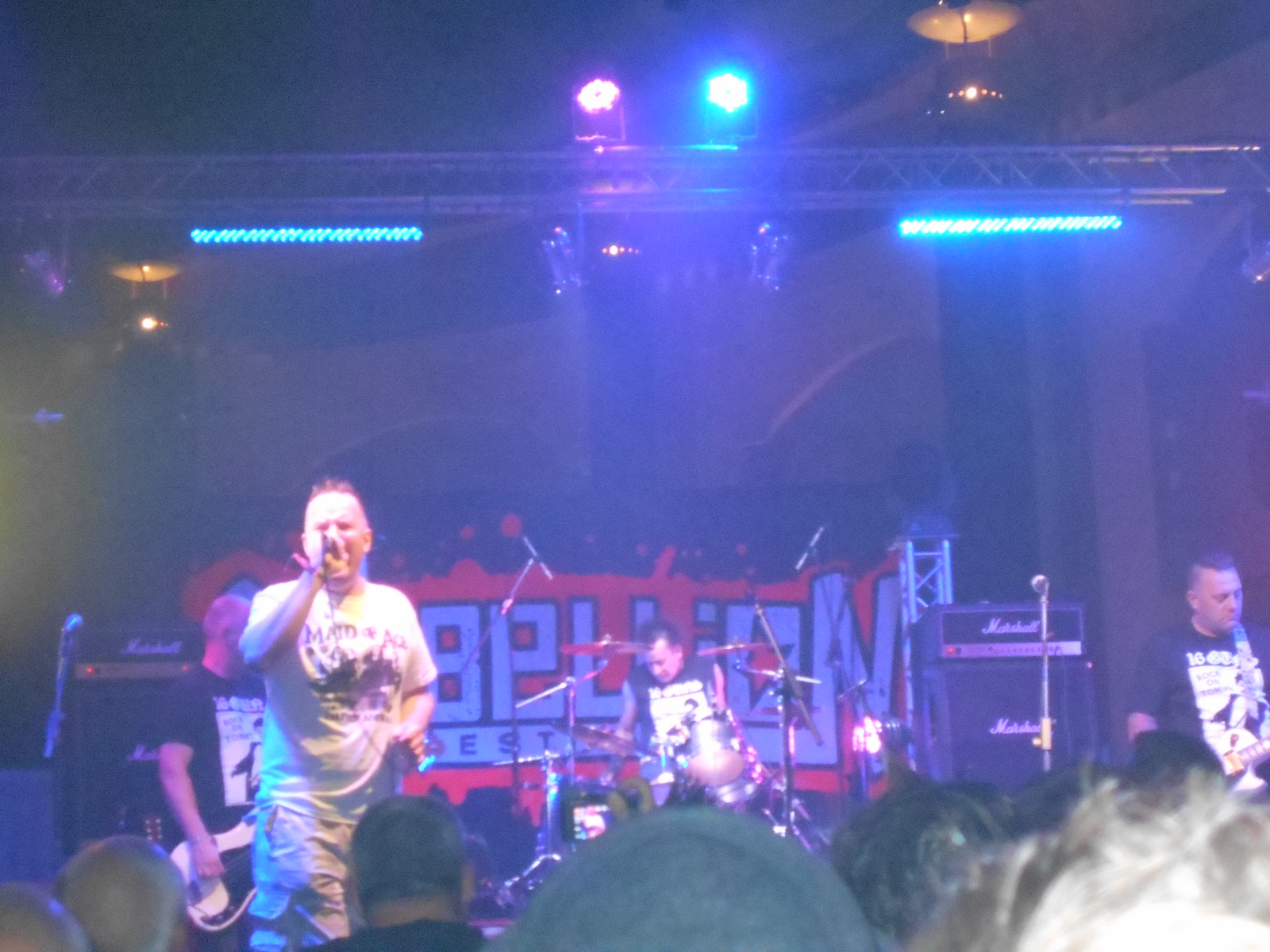The photograph captures a band mid-performance at a concert, with a mix of stage lighting contributing to the scene's dramatic feel. The setting is ambiguous, either interior or exterior, but the pitch-black backdrop leaves it unclear. Multiple lantern-style lights are suspended from various points, alongside blue and purple LED tube lights and two spotlights mounted on a metal scaffolding that resembles a ladder, built above the stage. The band comprises four members, all partially obscured by the heads of the audience visible at the bottom of the image.

The singer stands prominently in the foreground, sporting a white t-shirt with an indistinguishable black graphic, and is mid-song with a microphone raised to his mouth. He has almost bald hair, with some spiky hair on top. Behind him to the left, one guitarist is playing, dressed in a black t-shirt with a white graphic, and has his head sides shaved. Another guitarist, positioned on the far right, is similarly dressed in a black t-shirt with white design. Centered in the background is the drummer, identifiable by his black and white tank top and short brown hair. Behind the drummer, a sign reads "Rebellion" in large white letters, though partially obscured. The band members in black t-shirts appear to be wearing matching shirts, with the drummer's either having cut-off sleeves or rolled up. The atmosphere is lively, despite the slight blurriness of the image and the washed-out effect from the stage lighting.